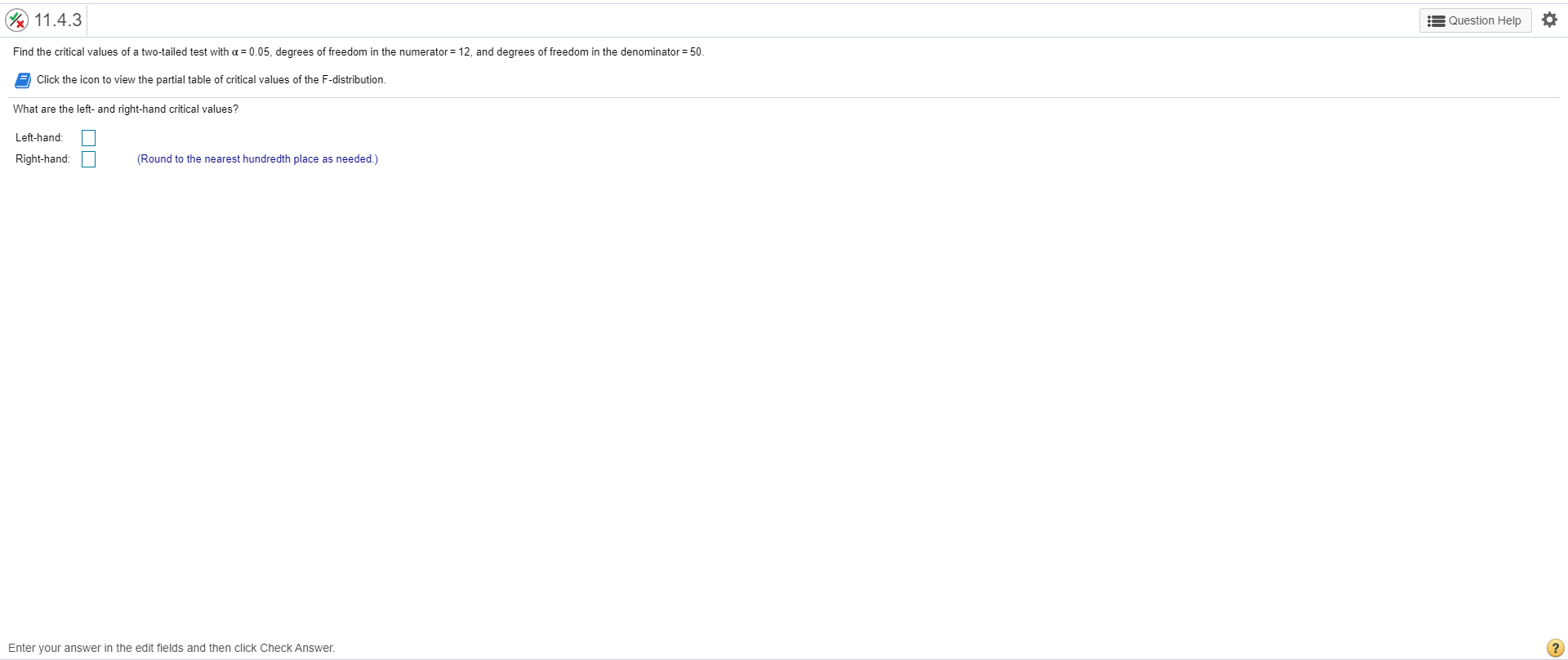**Caption:**

The image depicts an online quiz interface, possibly designed for educational purposes, such as assessing students' knowledge. The text on the screen is relatively small and challenging to read. In the top-left corner, there is a small logo featuring a green check mark over a red X, likely symbolizing correct and incorrect answers. Adjacent to this logo, the numbers "11.4.3" are displayed.

Directly below, the screen displays a question that reads, "Find the critical values of a two-tailed test with an alpha value of 0.05, degrees of freedom in the numerator equals 12, and degrees of freedom in the denominator equals 50. Click the icon to view the partial values of critical values of the F distribution." The text instructs users to click an icon represented by a blue book, situated to the left of the instruction.

Following the instruction to click the icon, the actual question is presented: "What are the left-hand and right-hand critical values?" There are input fields provided for users to enter these values, accompanied by blue text that instructs, "Round to the nearest hundredth place as needed." Below the left-hand input field, there is a second field for the right-hand prompt.

At the bottom-left of the screen, there's a note that says, "Enter your answer in the edit fields and then click check answer." On the bottom-right, a yellow question mark icon is visible, possibly offering assistance. The top-right features a gear icon for settings, and just left of it is the "Questions Help" button, available for additional guidance.